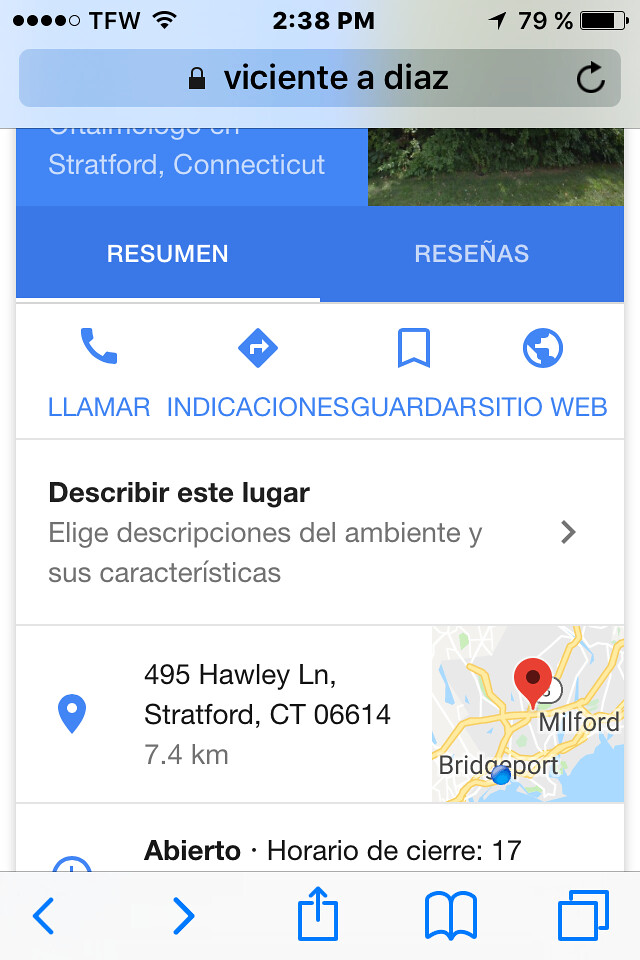This image is a screenshot taken from an iPhone, evident from the characteristic iPhone interface elements such as the digital clock centered at the top, battery percentage indicator, location services icon, Wi-Fi strength signal, and weather symbol. The primary content of the screenshot is a Google Maps display targeting the address 495 Holly Lane in Stratford, Connecticut. The map features a red dropped pin marking the specific location and a blue dot indicating the user's current position. Additional map details are predominantly displayed in Spanish, providing geographical context and navigational assistance within the app.